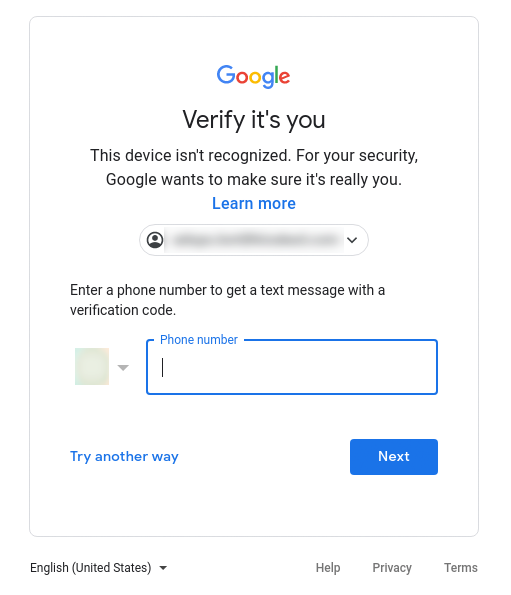The image depicts a Google verification pop-up message designed to confirm the user's identity for security purposes. The dialog box is a white, vertically elongated rectangle displaying the Google logo at the top. The logo features the letters "G" in blue, "O" in red, "O" in yellow, "G" in blue, "L" in green, and "E" in red.

Beneath the logo, the message reads, "Verify it's you. This device isn't recognized. For your security, Google wants to make sure it's really you." To the right of this text is a person icon enclosed in a circle, but the associated information has been blurred out. 

Below the verification notice, instructions prompt the user to "Enter a phone number to get a text message with a verification code." A tan-colored drop-down menu appears to be for selecting the country code. Adjacent to it is a blue-outlined field labeled "Phone number," which is currently empty and white.

At the bottom of the pop-up, there are two options: "Try another way" written in blue on the left, and a "Next" button in white on the right. A gray border encases this entire section of the dialog box.

Directly below the gray-bordered area, another section includes a drop-down menu on the left labeled "English (United States)," and on the right side of the same row, links for "Help," "Privacy," and "Terms" are displayed.

Overall, the image uses a color palette of blue, red, yellow, green, black, gray, and white.